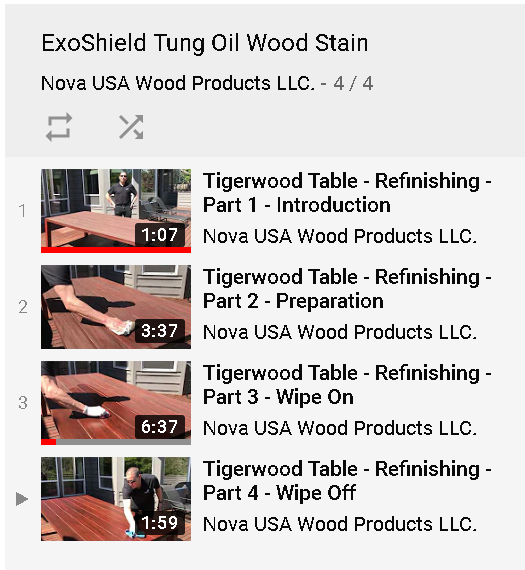This detailed caption clearly describes the elements in the image, providing all necessary context:

"The screenshot depicts a YouTube-like interface showcasing different methods of staining a table with Exoshield Tongue Oil. The top header, thicker than usual, features an off-white background with the text: 'Exoshield Tongue Oil Wood Stain' followed by 'Nova USA Wood Products LLC 4/4.' To the right, two buttons appear—a refresh button and another resembling an X made of two arrows. Below the header, there are thumbnails for four videos listed sequentially, each relating to the refinishing of a Tigerwood table. 

1. 'Tigerwood Table Refinishing Part One: Introduction' by Nova USA Wood Products LLC
2. 'Tigerwood Table Refinishing Part Two'
3. 'Tigerwood Table Refinishing Part Three'
4. 'Tigerwood Table Refinishing Part Four' - this one displays a play button, indicating it is currently selected.

Each thumbnail shows a man; he is fully visible in the first and fourth thumbnails, and his arm is partially visible in the second and third thumbnails. The overall layout gives a comprehensive guide to the process of using Exoshield Tongue Oil for table refinishing."